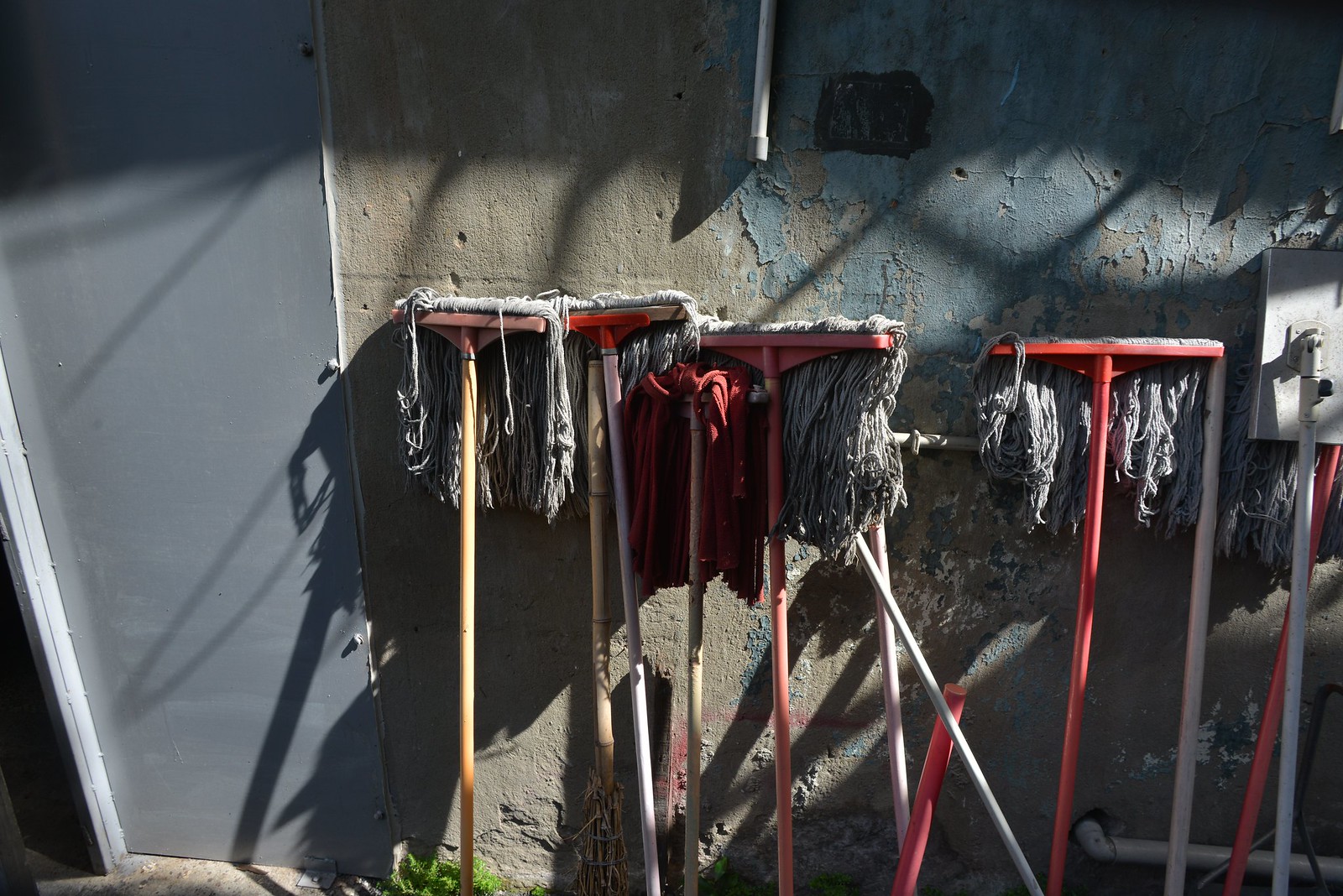The image captures an outdoor scene with a weather-beaten concrete wall, characterized by a rough stone brick texture and patches of faded, cracked blue paint. On the left side of the wall, a smooth gray doorway is partially visible, cut off by the edge of the image. Leaning against the wall are approximately eight mops, each with red plastic mop heads and worn, gray mop fibers that appear heavily used and dirty. The mop handles vary in color and material, including red, tan, metallic, and brown tones. Sunlight casts shadows across the scene, adding to the sense of an aged, sun-exposed environment.